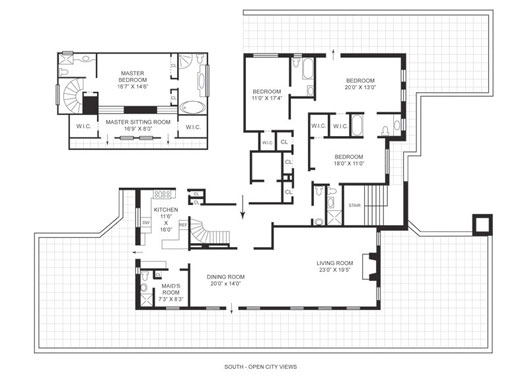This detailed, overhead blueprint illustrates a spacious multi-story house layout inked in black on a white background. The first floor consists of a 23' x 19' x 5' living room, a dining room, a maid's room, a kitchen, and three additional bedrooms. The largest of these first-floor bedrooms measures 20' x 13', accompanied by another at 11' x 17', and one at 18' x 11'. Notably, one of the first-floor bedrooms features two walk-in closets. Ascending the centrally located staircase leads to the second floor, where the master bedroom resides. The master suite dimensions are 16' 7" x 14' 6" and include two spacious walk-in closets and a dedicated master sitting room. The blueprint also partially outlines the lawn with a lighter design, accentuating the external boundaries. The walls are denoted with thicker lines to signify their structural significance, clearly distinguishing them from other elements in the blueprint.